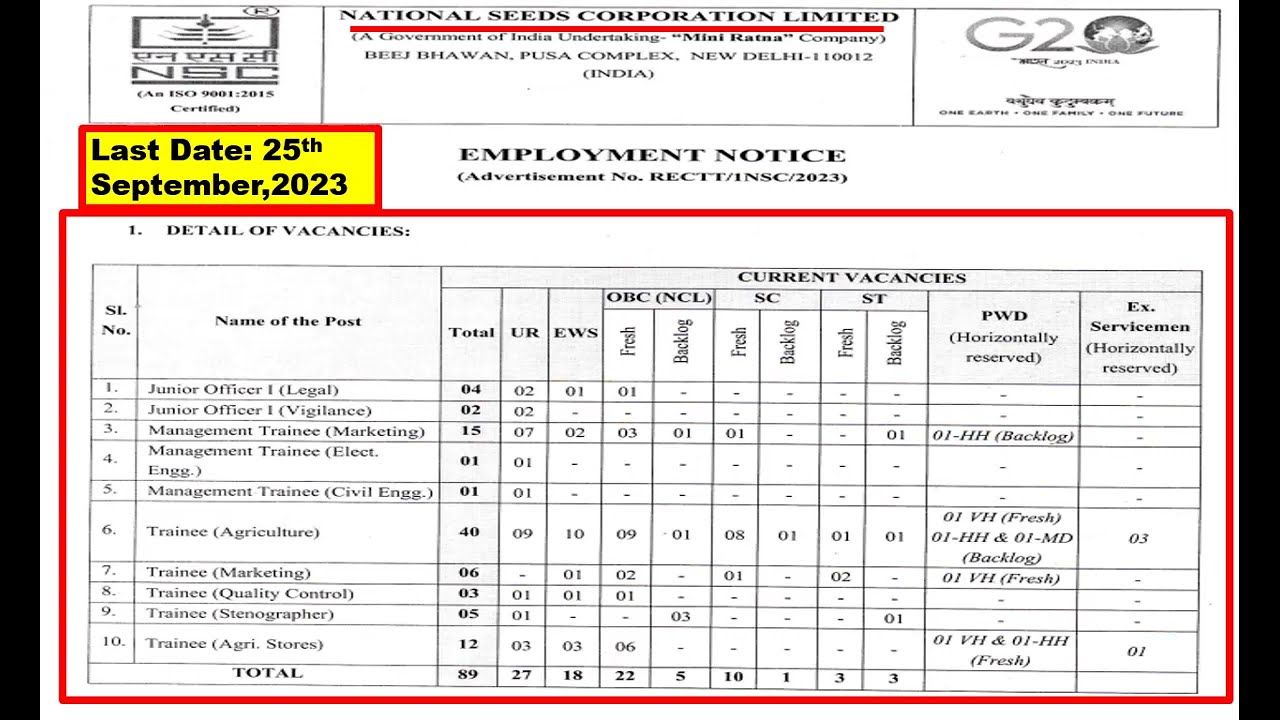This image depicts an employment notice from the National Seeds Corporation Limited (NSC). The notice is presented on a rectangular white piece of paper, roughly six inches wide and four inches tall, with black borders on the left and right sides. At the top left, there is a logo resembling a TV screen with the text "NSC," "ISO 9001:2015 certified" below it. The top middle prominently displays "National Seeds Corporation Limited" in bold black print, underlined in red. Below this, the text reads "A Government of India Undertaking," followed by "Mini Ratna Company Bij Bhawan, Pusa Complex, New Delhi 110012, India." The upper right corner features a G20 logo with the phrase "One Earth One Family One Future."

Adjacent to these elements, a yellow rectangle with a red outline states "Last date: 25th September 2023" in black print. To the right, "Employment Notice, Advertisement Number RECTT/1NSC/2023" is printed on a white background. Below, a large red-bordered table is titled "Details of Vacancies." This table organizes information into columns with headers such as "SL Number," "Name of the Post," "Total," "UR," "EWS," "OBC (NCL)," "SC," "ST," "PWD," and "Ex-Serviceman." The posts listed include "Junior Officer I," "Junior Officer I (Diligence)," "Management Trainee," and various trainee positions, providing detailed attributes and vacancies for each role.